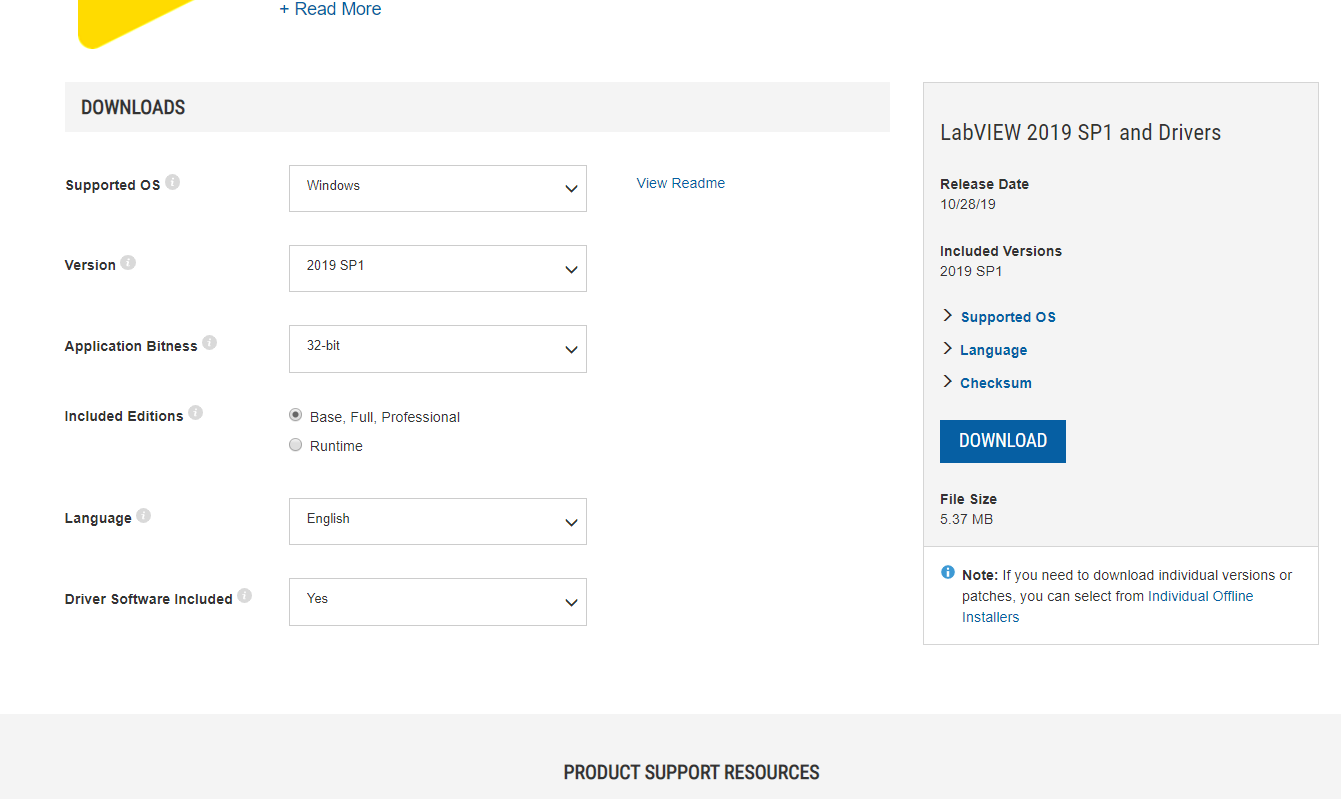Website Page Description:

The webpage features a predominantly white background, interspersed with a few off-white banners and bars. In the upper left corner, there is a small, uniquely shaped yellow logo, which is neither perfectly square nor round, but a blend of both shapes. Directly below this, a light gray bar is labeled "Downloads" in black text.

Below the Downloads bar, there are several options accompanied by drop-down menus. These options include:

1. Supported OS
2. Versions
3. Application Bitness
4. Included Editions
5. Language
6. Driver Software Included

On the right side of the webpage, there is a tall, rectangular box with a light gray background. The top of this box displays the text "LabVIEW 2019 SP1 and Drivers," followed by the release date "10-28-19."

At the very bottom of the page, another light gray rectangular box contains the text "Product Support Resources."